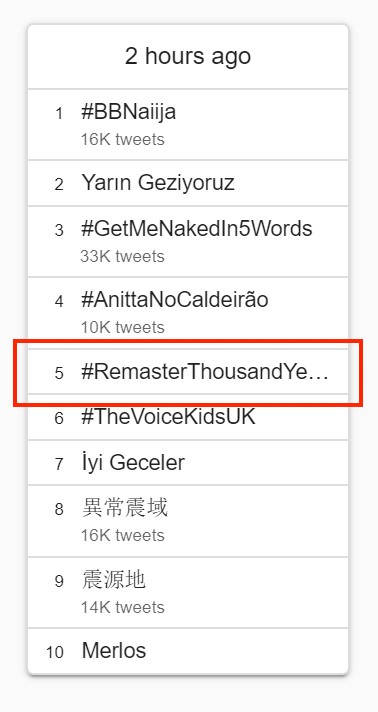This image is a screenshot of a numbered list ranging from 1 to 10, showcasing trending topics on a social media platform. The background of the list is a clean white, while the text is primarily black and gray. Each item on the list is separated by thin, light gray lines for clarity. At the top of the list, there is a header that reads "2h ago," indicating that the trends are from two hours prior.

1. **#BBNija**, 16k tweets
2. **Yerin Gezirutz**
3. **#GetMeNakedIn5Words**, 33k tweets
4. **#AnitaNoCalderao**, 10k tweets
5. **#Remaster1000Yi** (highlighted with a red rectangle)
6. **#TheVoiceKidsUK**
7. **AEGessler**
8. **Chinese Characters**, 16k tweets
9. **Chinese Characters**, 14k tweets
10. **Merlos**

The juxtaposition of various hashtags, names, and Chinese characters represents a diverse set of trending topics, with the special emphasis on item number 5, indicating it may have significant relevance or personal importance to the person who took the screenshot.